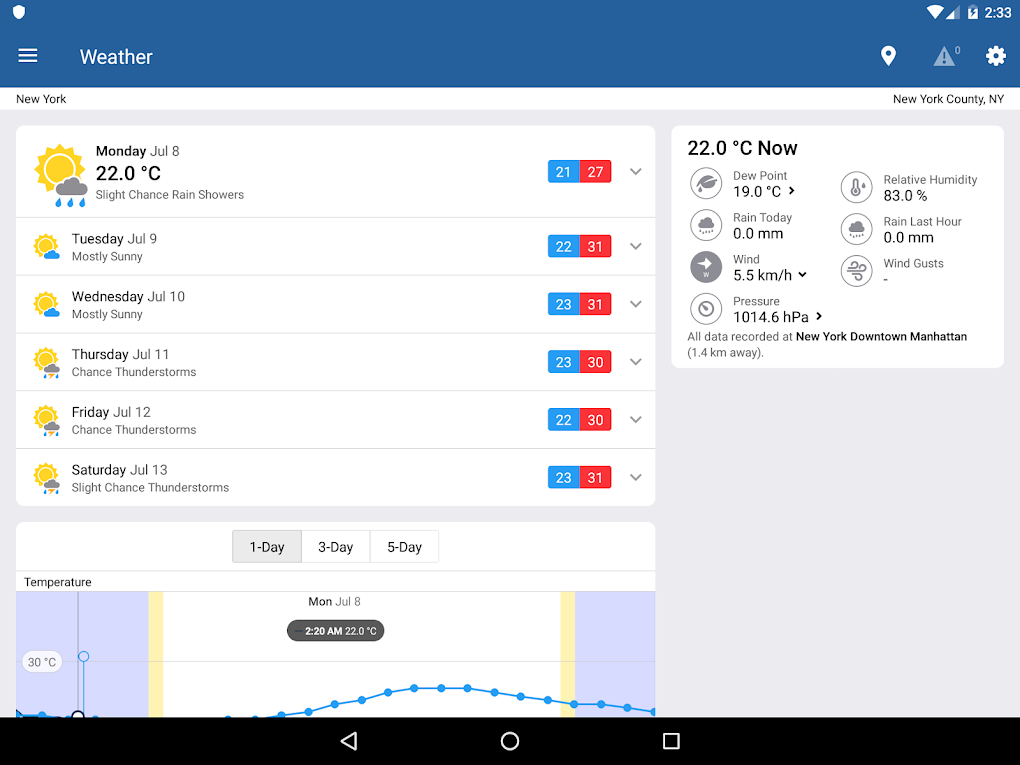This image depicts a screenshot from a weather application displayed on a tablet, as evidenced by the widescreen format and the presence of typical tablet navigation buttons, including the home, tab, and back buttons visible at the bottom of the screen. The application interface is topped with the simple heading "Weather," indicating it is providing meteorological information for New York County, New York.

The central part of the screen features a detailed weekly weather forecast, primarily showing sunny conditions interspersed with occasional clouds and rain. The forecasted temperatures range from lows of 21°C to highs of 31°C, highlighting a notable variation over the week.

On the right-hand side of the screen, additional meteorological data is presented, giving an in-depth look at current weather conditions. This includes the dew point, precipitation for the current day, wind speed, atmospheric pressure, relative humidity, rainfall in the last hour, and wind gusts. Additionally, the current temperature is indicated as 22°C.

At the bottom of the screen, there are options to view the weather data in graph form for different durations—one day, three days, and five days. The current selection is set to display the one-day graph, which charts the temperature variations throughout the day. The combination of these elements provides a comprehensive overview of the weather conditions and forecasts for New York County, New York.